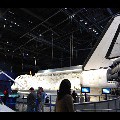This low-resolution thumbnail image appears to be set in a dark industrial or warehouse setting, potentially even a museum. Dominated by black borders at the top and bottom, much of the background remains shrouded in darkness, punctuated by small highlights and a strip of bluish-green light to the left-hand side. At the center of the image stands a white object with black and gray accents, likely a spaceship or airplane, given its visible wing extending towards the top right. Beneath the tail portion of this white craft, two bright blue lights glow prominently. Surrounding the object is a fenced area, within which three human figures are discernible. One individual, with dark long hair, stands in the lower center facing away, draped in a jacket. To this person's left stand two others, possibly observing the scene. Additional details include a small red dot and two bluish-whitish boxes or screens positioned towards the bottom right, further enriching the visual complexity of this intriguing, though diminutive, image.